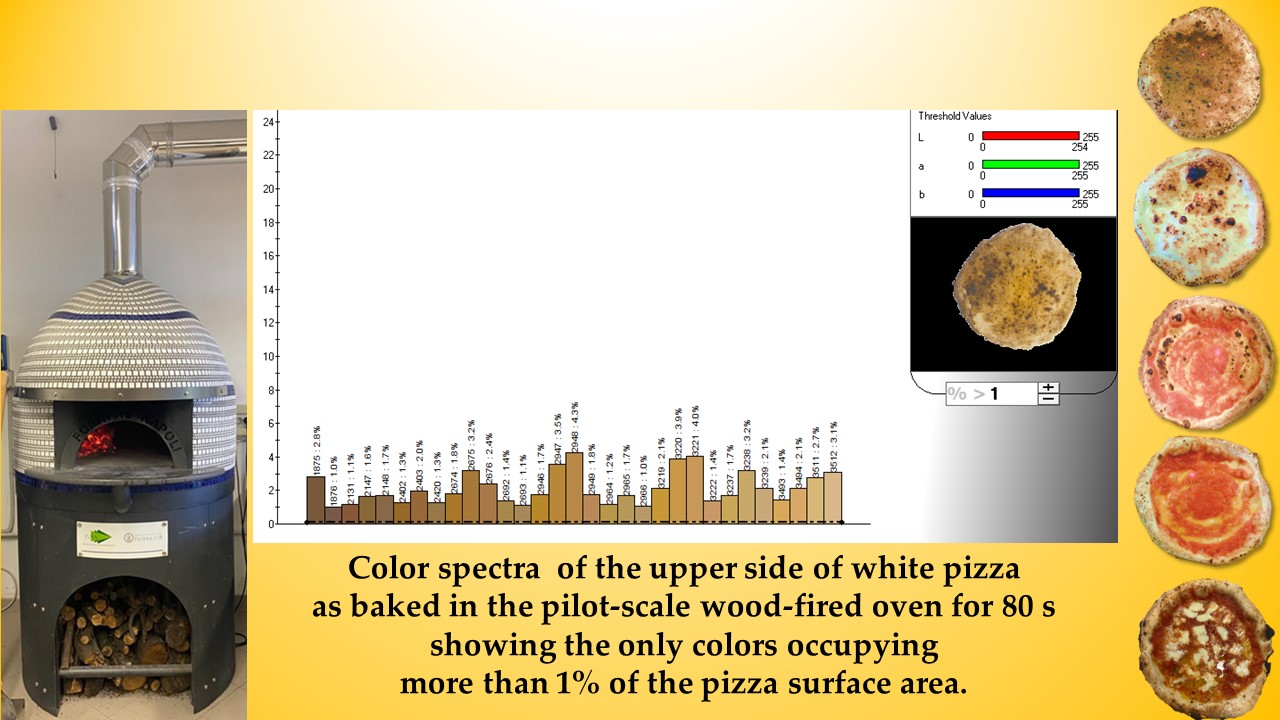The image showcases a detailed pizza-themed diagram centered around the cooking process and analysis of pizzas. On the far left, there's a photograph of a wood-fired pizza oven made of metal with visible bolts and an exhaust pipe, stacked on firewood. The oven has a reddish fire burning inside. To the right side of the oven, a series of photographed pizzas in varying stages of preparation are displayed: from loaded with sauces and cheeses at the bottom, progressively less saucy pizzas in the middle, to plain dough at the top. Dominating the central portion of the image is an informative bar chart depicting the color spectra of the upper surface of a white pizza baked in a pilot-scale wood-fired oven for 80 minutes. The chart includes bars for red, green, and blue values, and explains that these colors occupy more than 1% of the pizza surface area. There are numerical notations and LAB values correlated with the bar graph, which is presented on a clean white backdrop, making the threshold values easily readable. The entire setup suggests a comprehensive analysis of pizza baking, likely excerpted from an instructional manual or a detailed pizza study.